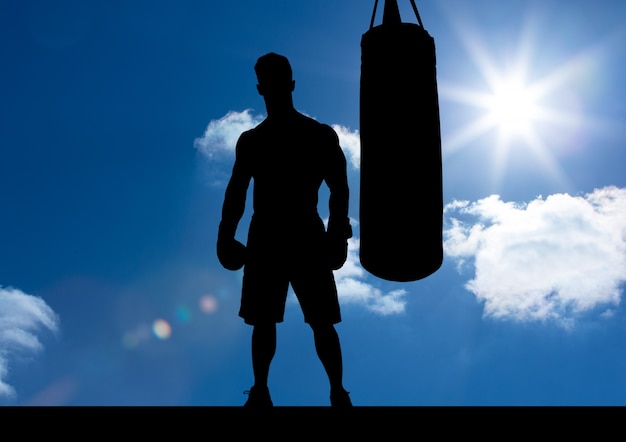In this striking image, the foreground features a powerful silhouette of a heavily muscled boxer donning boxing gear, which includes gloves, trunks, and boots. He stands resolutely on a flat, indiscernible surface, with a punching bag hanging beside him. The silhouette is rendered in deep black, obscuring specific facial features and leaving him almost shadow-like. The bright Sun dominates the top right-hand corner, radiating a noticeable starburst effect that adds a dramatic lens flare across the scene. The backdrop is a vivid blue sky scattered with fluffy white clouds, creating a stark contrast against the dark foreground figures. The detailed starburst effect from the Sun spreads diagonally downward, intersecting the boxer's right leg and the punching bag, casting ethereal streaks of blue, pink, and yellow light. Clouds are dispersed across the sky, one prominently positioned on the bottom left and another large one occupying much of the middle right area of the image. The composition presents a dynamic interplay between light and dark, emphasizing the boxer's poised stillness against the vibrant, sunlit sky.